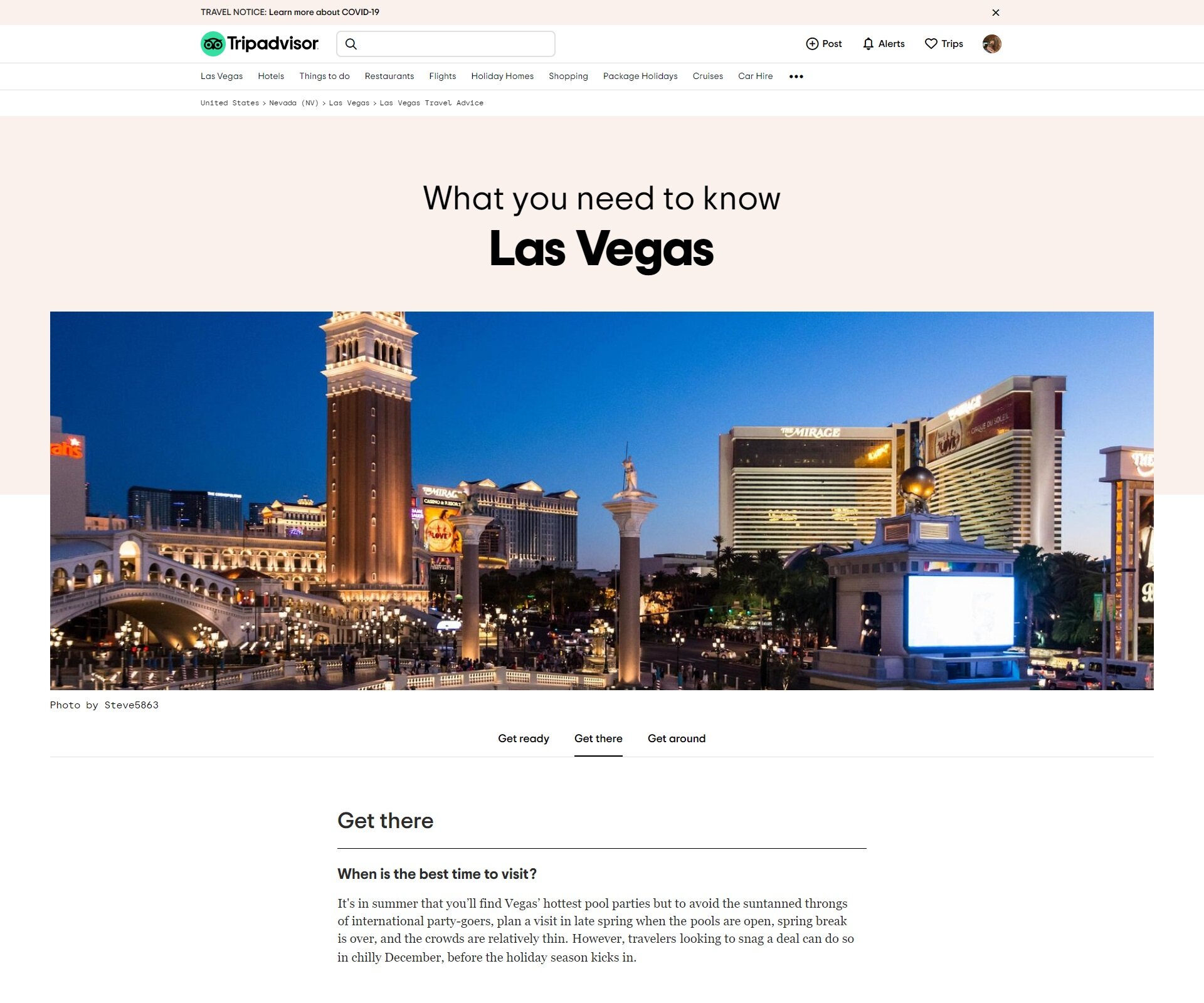The screenshot captures a TripAdvisor webpage, prominently featuring the TripAdvisor logo at the top left, complete with its distinctive green icon that includes a stylized owl. The background is a mix of beige and white tones, providing a neutral backdrop for the content. 

Central to the page is a bold black heading: "What You Need to Know - Las Vegas." Underneath this heading is an eye-catching photograph of the Las Vegas skyline, dominated by a vibrant display of illuminated buildings and iconic landmarks. On the left side of the image, a towering structure and an archway catch the eye, while skyscrapers rise prominently in the background. The right side of the photo showcases The Mirage, with its large, illuminated sign and an adjacent white screen. The sky above transitions from a dark, almost nighttime hue on the left, to a lighter tone on the right, suggesting dusk.

Beneath the photograph, informative text is displayed, beginning with a prompt: "Get There." It goes on to offer advice on the best time to visit Las Vegas. The text notes that summer is ideal for experiencing the city's hottest pool parties. However, for those looking to avoid the bustling crowds, late spring is recommended, with open pools and the end of spring break resulting in thinner crowds. Additionally, budget-conscious travelers might consider visiting in chilly December, prior to the holiday season, for potential deals.